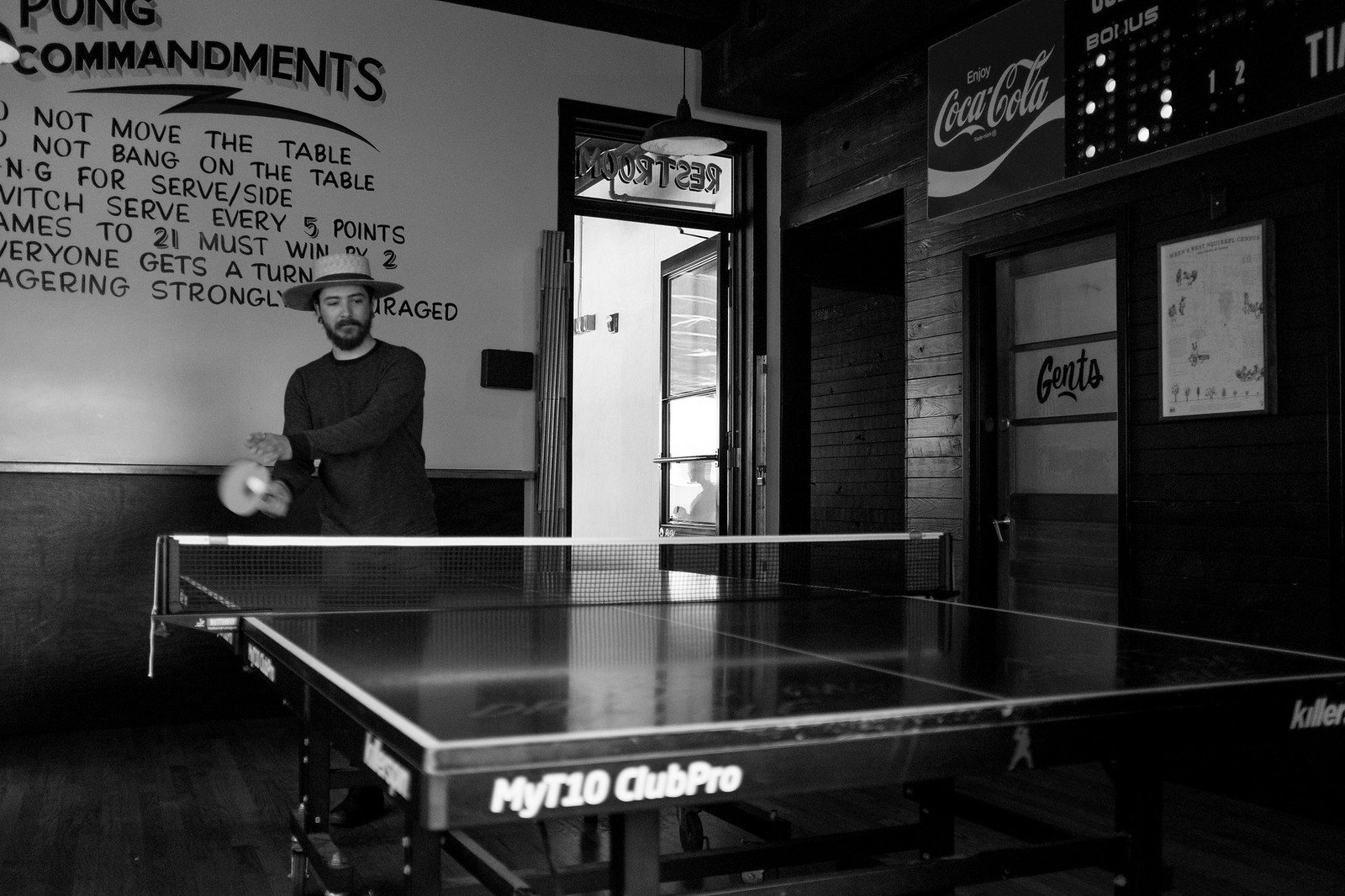The black and white photograph appears to capture a contemporary scene, framed with the nostalgic aesthetic of an older era. It depicts an interior space of a bar, characterized by brick and hardwood walls. A worn-out Coca-Cola sign and a hand-painted restroom door labeled "Gents" complement the rustic ambiance. 

Central to the image is a ping-pong table, with prominently visible text on the side that reads "My T10 Club Pro." The perspective of the shot is a close-up view from the end of the table. Positioned just left of center is a light-skinned man in his late 20s or early 30s. He sports a hipster-style black beard, a white wide-brimmed hat, and a long-sleeved gray shirt. Captured in mid-motion, the man is in the act of serving a ping-pong ball, which is frozen in a blur just off his paddle as he looks down at the table with focus.

Adorning the wall behind him is a prominently displayed, hand-painted list titled "Ping-Pong Commandments." Despite being partially obscured by the frame, the visible rules advise: "Do not move the table," "Do not bang the table," "First serve/side," "Switch serve every 5 points," "Games to 21, must win by 2," and "Everyone gets a turn, wagering strongly encouraged." This meticulous detailing suggests a ping-pong section within the bar, lovingly curated for leisure and competition.